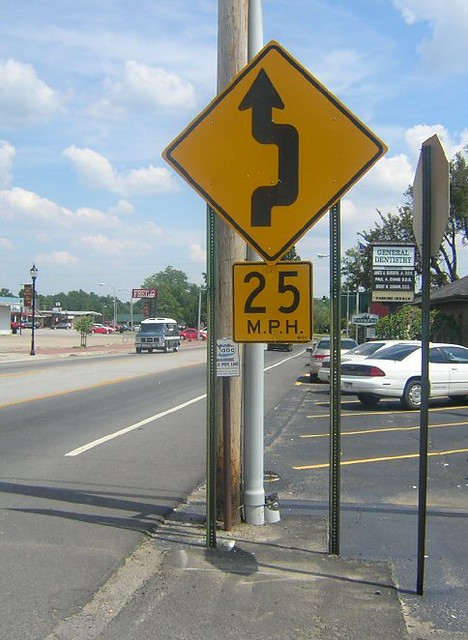The image captures an outdoor scene dominated by a partly cloudy sky, where patches of blue peek through white clouds. Centrally featured are two road signs. The upper sign is diamond-shaped with a black border and contains a black, squiggly arrow pointing upwards, signaling a winding road ahead. Directly below this, a smaller, square-shaped sign indicates a speed limit of 25 mph, with "m.p.h" clearly written in black. In the background, several cars are visible, some of which are parked, adding context to the roadside setting.